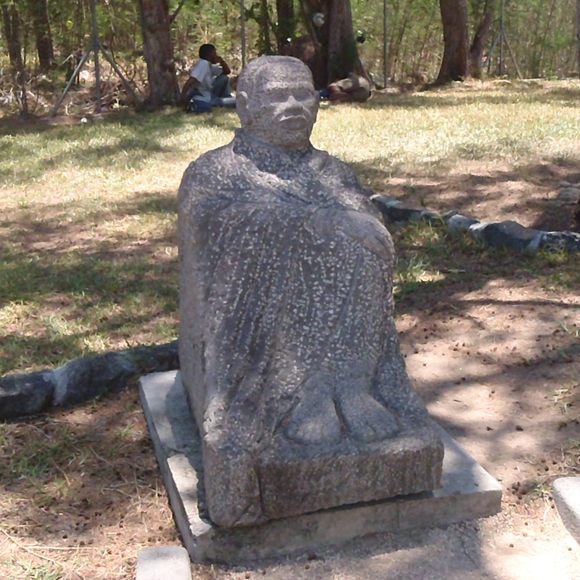The image showcases a detailed stone statue of a man seated on a small concrete slab in what appears to be a public park. The man in the statue, possibly of African descent, is depicted sitting with his legs pulled up to his chest and arms wrapped around his knees, covered in a cloak or blanket that leaves only his head, hands, and feet visible. The statue is crafted from granite stone, displaying varying shades of grey and white from chipping. Surrounding the statue, the ground transitions from soil to dry grass, indicating a late summer or early autumn setting. Behind the statue, a ridge made of rocks can be seen, leading to more dry grass. Further in the background, a person of African descent is sitting on the grass, relaxing in the park. The scene is framed by trees and a greyish wire fence, with additional trees beyond the fence, suggesting a wooded area.